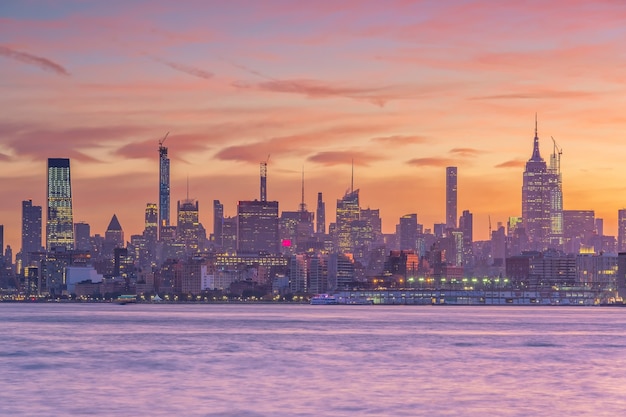The photograph captures a stunning cityscape at sunset, with a mesmerizing sky painted in hues of blue, pink, and orange, accentuated by light orange clouds. The city skyline features a myriad of tall, mostly grey buildings, with many windows illuminated, suggesting evening time. Some skyscrapers are adorned with cranes and scaffolding, hinting at ongoing construction. The midground reveals a well-lit pier and shore, where boats are docked. In the foreground, calm light blue and white water, devoid of waves, separates the viewer from the city. Trees dot the middle left and center of the image, adding a touch of nature to the urban scene. The concrete embankments along the shoreline frame the tranquil waterway, completing the picturesque view.